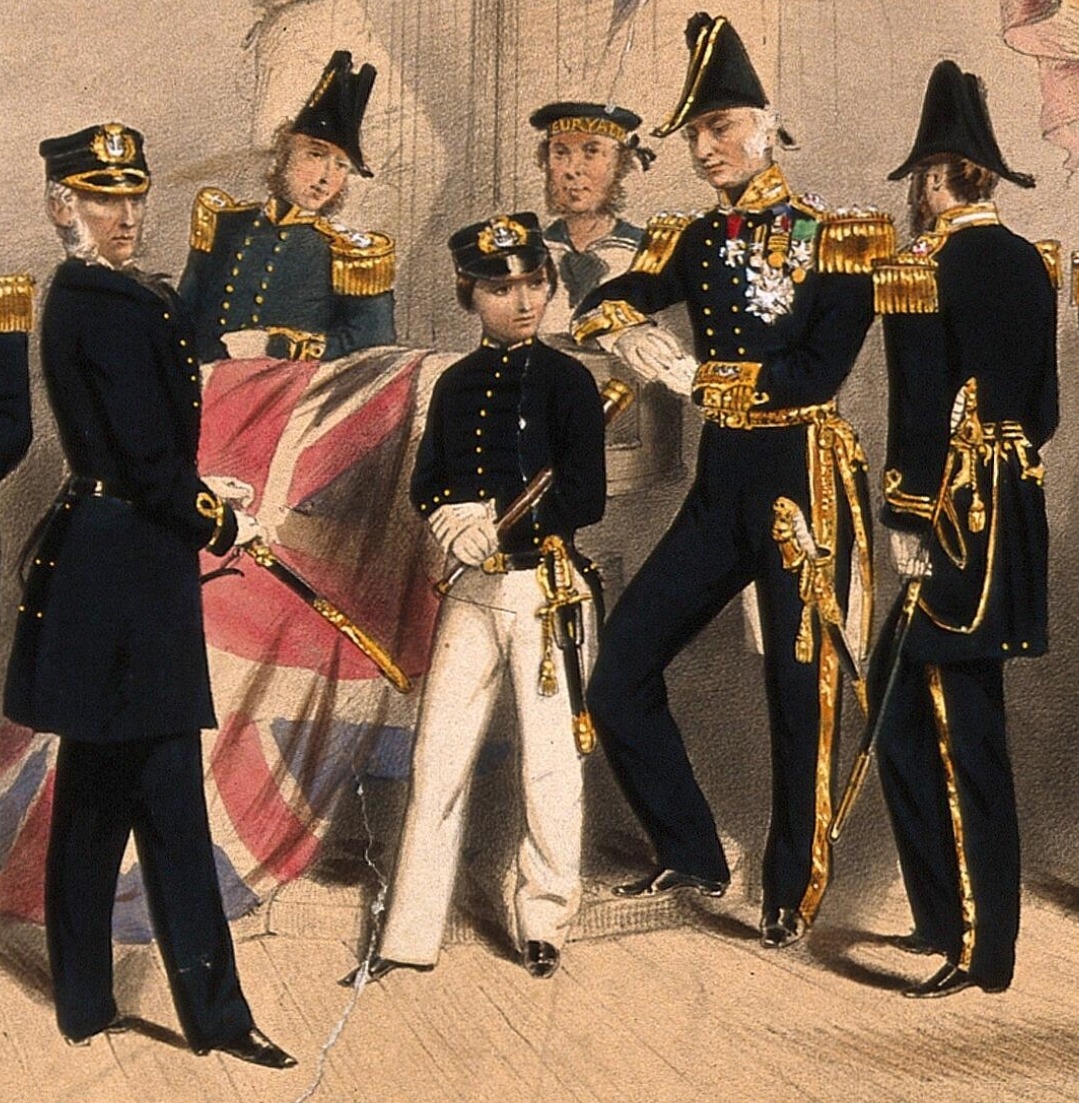This image depicts an old-time painting capturing a scene with six individuals, likely military personnel, adorned in elaborate, period-specific attire. The composition, slightly taller than it is wide, situates the figures against a beige-colored interior. Central to the scene is a young boy dressed in a black buttoned jacket and white pants, holding what appears to be a telescope. His outfit includes a black hat and black pointy shoes, common elements among the group. Flanking him are men dressed in distinguished black uniforms, each detailed with gold accents, embroidery, and various badges. Noteworthy among these figures are a man with white hair and mutton chops bearing a sword, a man with a tri-corner hat, and another in a similar black military dress.

On the left side of the image, two figures stand out. One, in a black military dress, appears to be holding a tattered British flag, and another positioned behind him dressed in a different greenish-blue uniform with golden tassels. A man at the back, possibly a sailor given his white and blue attire, completes the group. Each individual’s attire and the inclusion of elements like swords, scabbards, and possibly sabers hint at their military status, while the golden tassels and embroidery signify their ranks or roles. The flag, identified as the Union Jack, further anchors this scene in a historical, possibly British, military context.